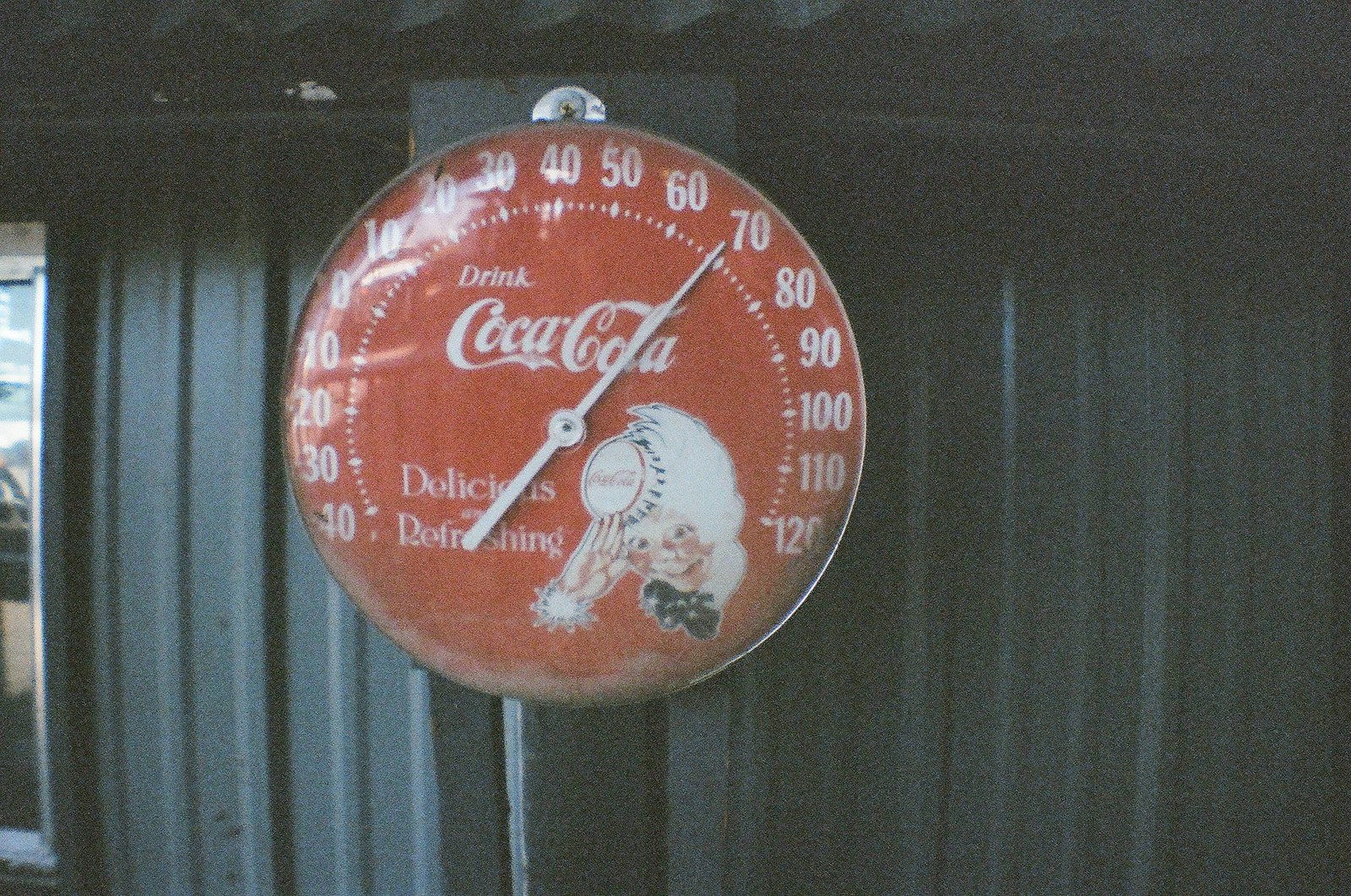The focal point of this image is a vintage Coca-Cola temperature gauge, typically found outdoors. The gauge, featuring an older style, is predominantly red and fastened to a pole. In the background, there's a metal building with a dark evergreen color, partially framed by a window to the left.

Central to the gauge's design is the iconic "Drink Coca-Cola" slogan displayed in the traditional Coca-Cola font, with white lettering set against a red background. Below the slogan, there's an illustrated character with white hair wearing a white bottle cap emblazoned with "Coca-Cola" in red letters. The character, dressed in a blue bow tie, appears to be in a saluting gesture. Adjacent to the character, the phrase "Delicious and Refreshing" is written in white letters.

The temperature readings on the gauge range from -10 degrees to 120 degrees Fahrenheit, with the numbers arranged around three-quarters of the circle, starting from -10 degrees on the left side and progressing clockwise.